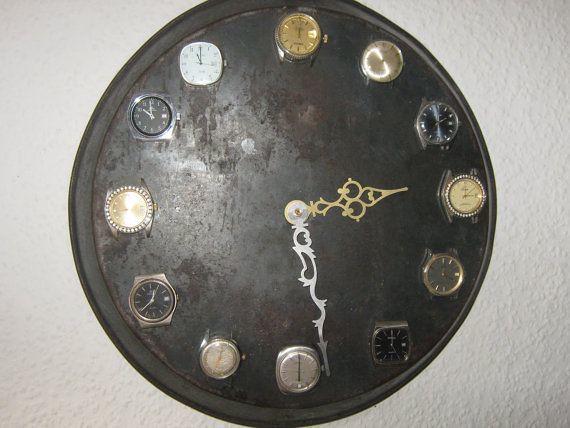This photograph features a distinctive wall clock hanging on a textured white wall. The clock's face showcases a creatively rusted metal background, reminiscent of a weathered pizza pan. Instead of traditional numbers, each hour is marked by a unique watch face—ranging in color and design, including a gold watch face at the 12 o'clock position, a lighter gold, shiny face at 1 o'clock, and a navy blue face at 2 o'clock. The 4 o'clock watch features a diamond bezel with a cream-colored face, while both the 3 and 9 o'clock positions also boast diamond bezels. The watch faces vary in shape from round to oval and square, with colors including black, light gray, yellow, white, and silver. The clock’s hands are intricately carved, with the shorter hour hand made of gold, and the longer minute hand made of silver, each adorned with elegant designs that taper into points. These hands are pointing towards the 3 and 6 positions, respectively, adding to the clock's elaborate and artistic appeal.